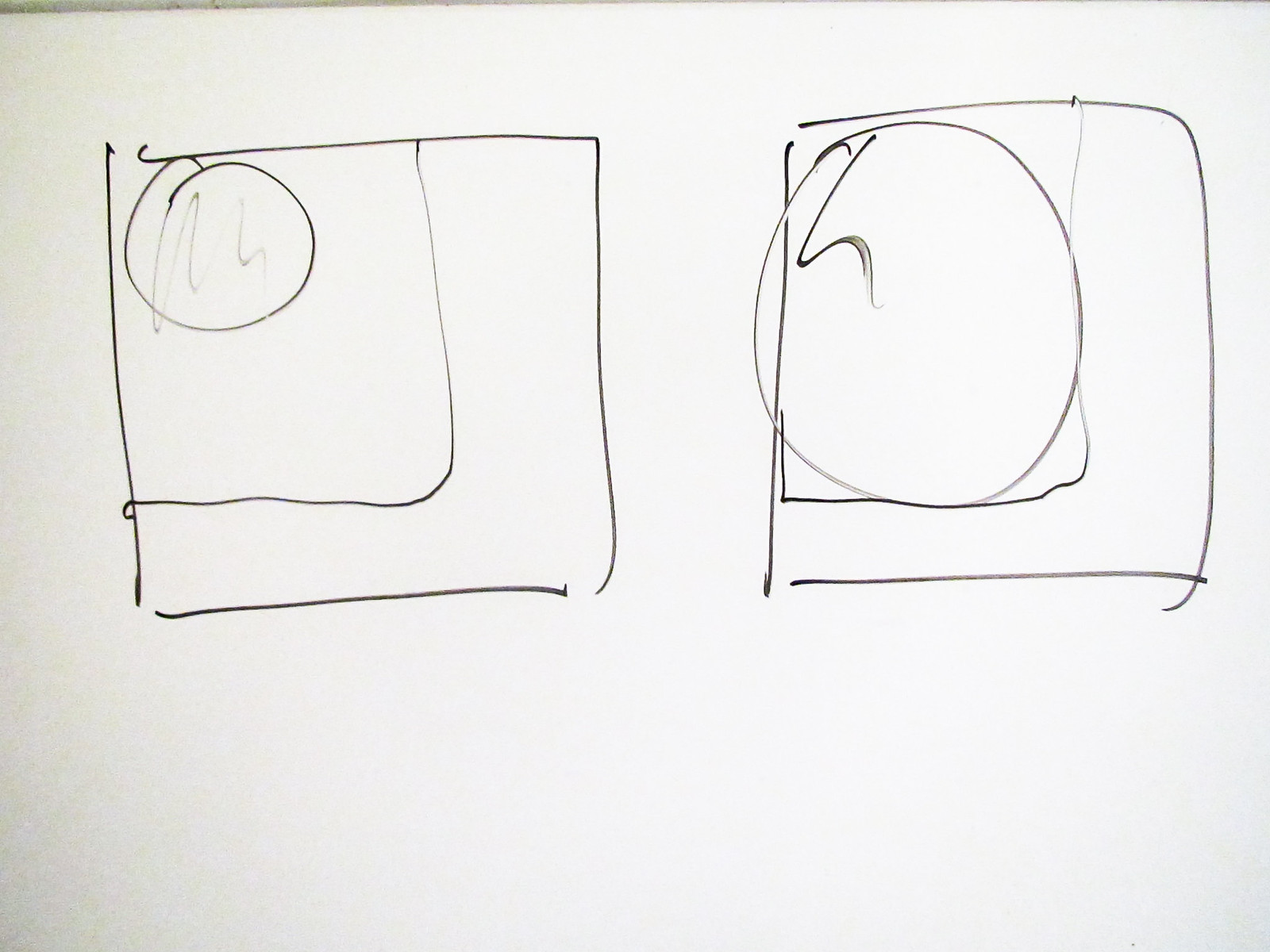This image showcases a drawing on a large, blank white sheet of paper, featuring two adjacent squares crudely sketched in either pen or marker. The square on the left contains an inner, slightly smaller square with an L-shaped line extending to the left. In its upper left corner, there's a circle with an indistinct mark or possibly an "H" inside. The right square mirrors the left, with a proportional smaller square inside; however, unlike its counterpart, this inner square is completely filled with a circle. The drawing's lines are inconsistent, with some not fully connected and little swirls at certain edges. The rest of the sheet remains empty, except for a faint sliver of something partially visible behind the paper in the upper left corner. The varying intensity of the lines adds to the drawing's crude and abstract nature.